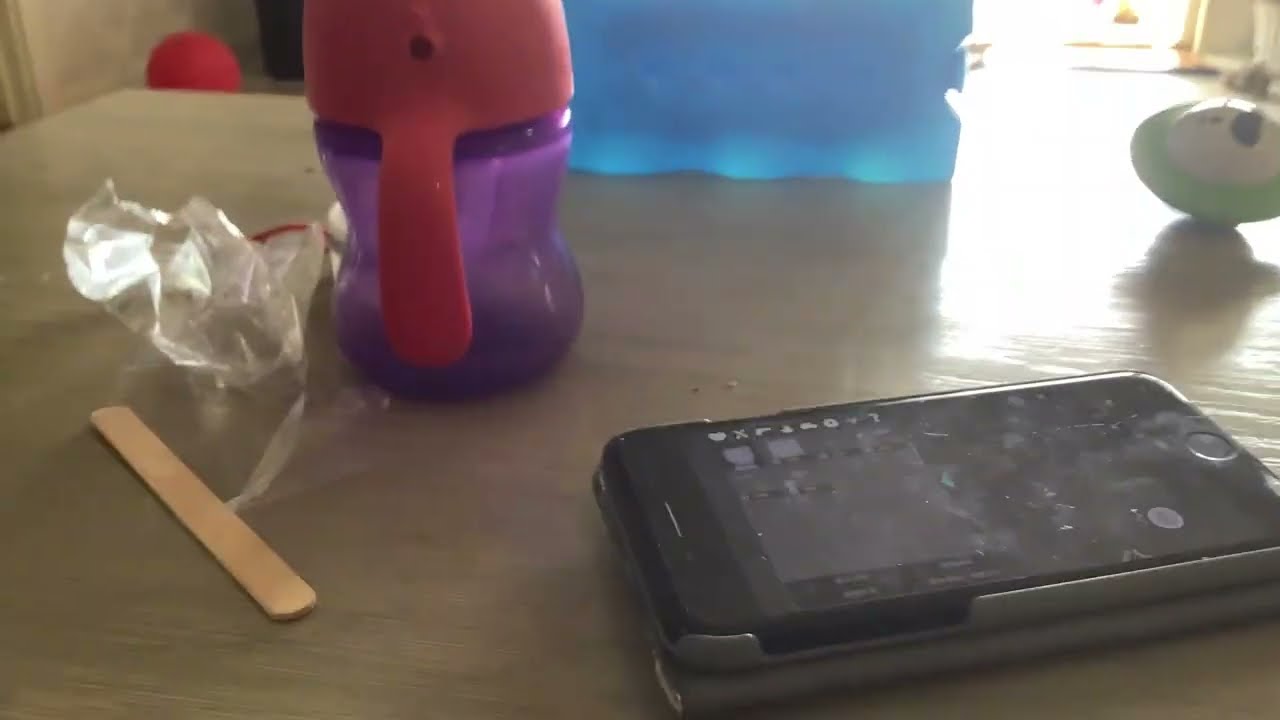This is a photo of a light wooden table scattered with various objects. In the foreground, the bottom right corner features an iPhone with its screen facing up, encased in a protective cover. Adjacent to the phone is a charger. Towards the left, there is a wooden Popsicle stick accompanied by a crinkled, clear plastic wrapper. Above these items, a child’s sippy cup with a purple base and pink lid, complete with a side handle, is prominently placed. Behind the cup, a blue square-shaped freezer container, typically used for ice or lunch boxes, is visible. In the background on the right side of the photo, partially cropped off, is a little green oval toy. Additional small details include a red ball against the wall in the upper left corner and a spinning top in the upper right corner.